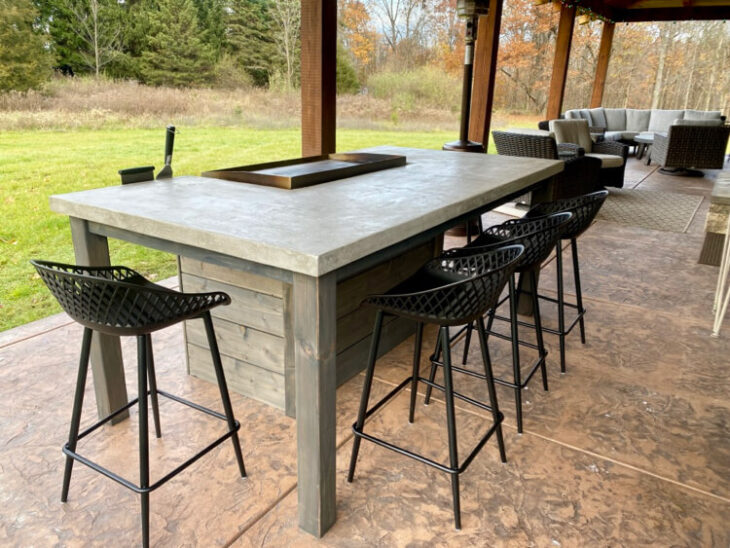This photo captures a cozy outdoor seating area, likely in someone's backyard, featuring a spacious grey stone table with a built-in fire pit in the center. The table, supported by rectangular legs, is surrounded by tall, short-backed black stools. Overhead, an awning supported by rectangular brown posts offers protection from the elements. To the right, there are a large grey sectional couch and additional grey chairs, providing ample seating. Beyond the seating area, a well-maintained lawn stretches out towards a backdrop of large, green evergreen trees and some bare deciduous trees, with hints of yellow leaves. The overall setting combines function and comfort, making it an inviting space for outdoor gatherings.